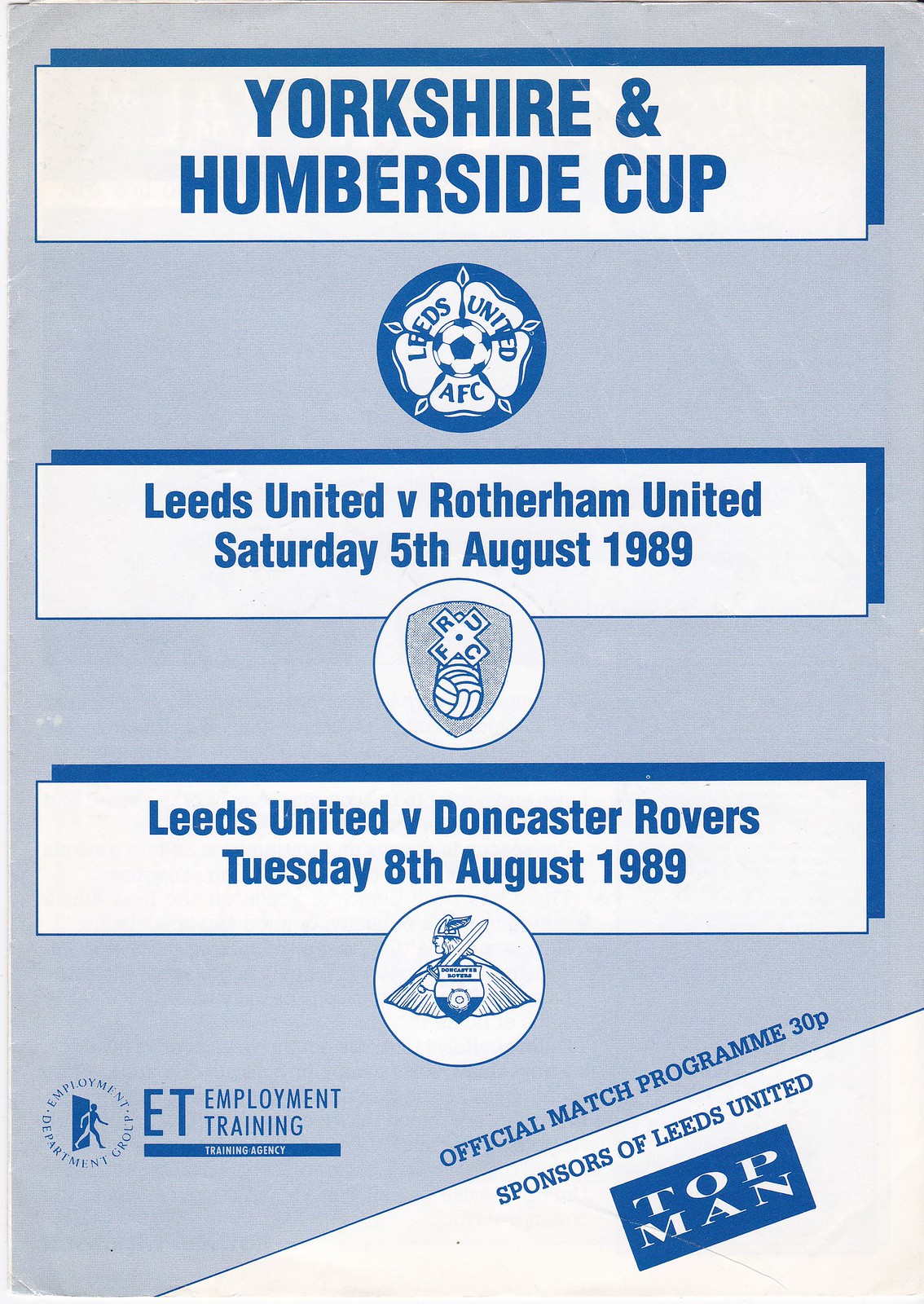The image is of a pamphlet on light blue paper, printed with dark blue and white text. Its content is organized into three sections. At the top, the pamphlet title "Yorkshire and Humberside Cup" is displayed in dark blue font. Directly below, there is a logo for Leeds United AFC, featuring a soccer ball encircled by petals resembling a flower. The pamphlet details matches, beginning with "Leeds United vs. Rotherham United, Saturday, 5th August 1989." Following this text is a logo for RUFC that includes a shield with a soccer ball and a crossed 'X.' Below, it announces "Leeds United vs. Doncaster Rovers, Tuesday, 8th August 1989," accompanied by another logo of a warrior figure in a winged helmet, holding a sword. The bottom section notes "Employment Training Agency, Official Match Program, 30P, Sponsor of Leeds United, Topman," with corresponding logos in white. The pamphlet has additional white accents, including a corner or border area.